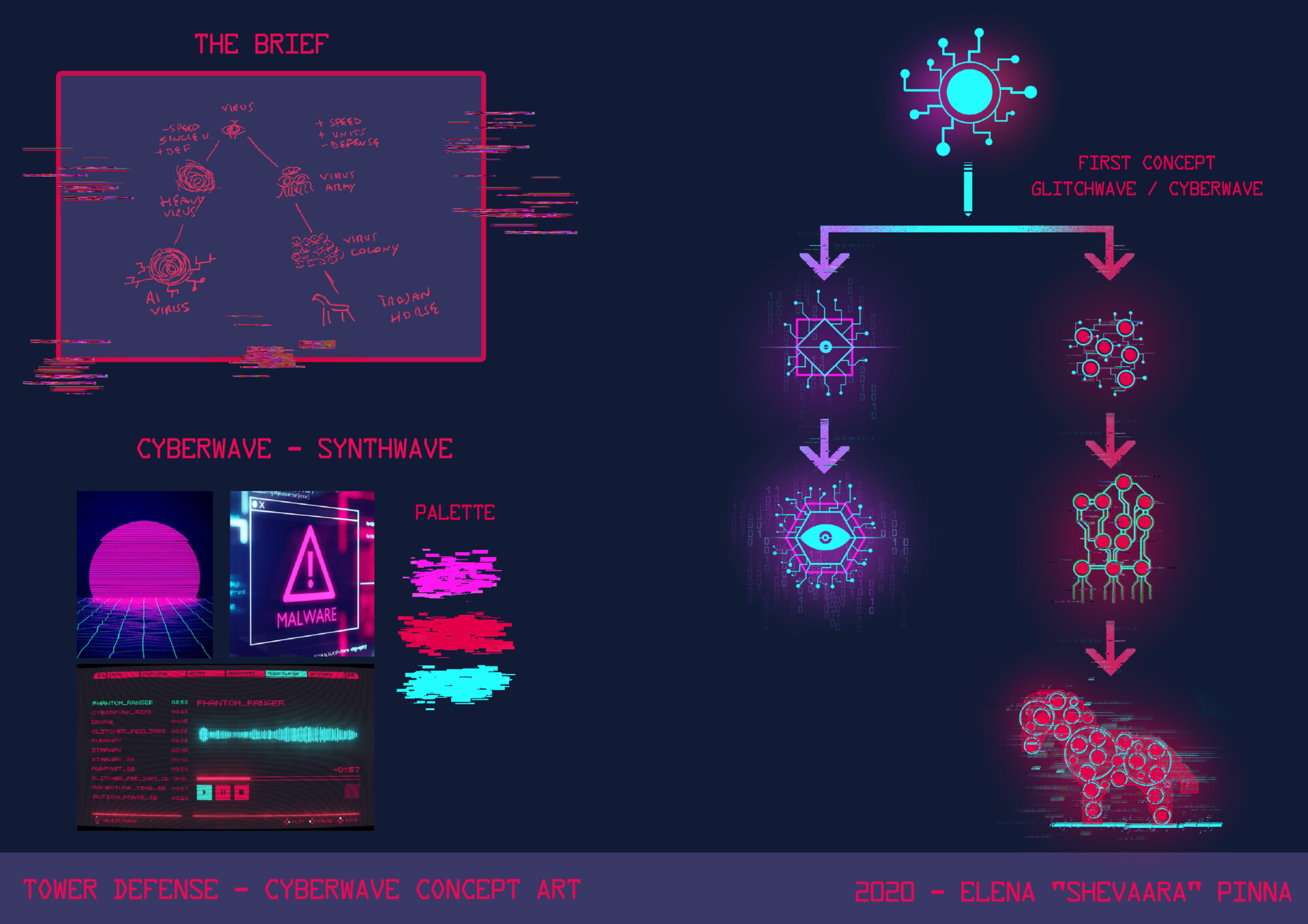This is a multicolored digital artwork, square in format, most likely extracted from a computer interface or video game concept. The overall background is essentially black, potentially with hints of navy blue. The piece features a variety of colors including pink, purple, and light blue. 

Prominently, there is a pink-outlined box with a lighter gray background in the center. Inside this box, tiny drawings and red digital text are present, although the text is too small to read. In the upper left corner of the image, in red text, it reads "The Brief". Directly below this, in red text as well, the words "CyberWave - Synthwave" are printed.

On the right side, a light blue circular image with small legs and dots, akin to a stylized electronic component, is connected by arrows pointing towards purple and pink images. At the bottom of the box in gray, detailed drawings form what appears to be an outline of a horse composed of circles. 

A dark gray border runs along the bottom of the piece, containing text in dark pink that reads "Tower Defense - CyberWave Concept Art 2020". On the far right side of this border, it states "2020 - Elena 'Shivara' Pina" accompanied by a collection of electronic symbols.